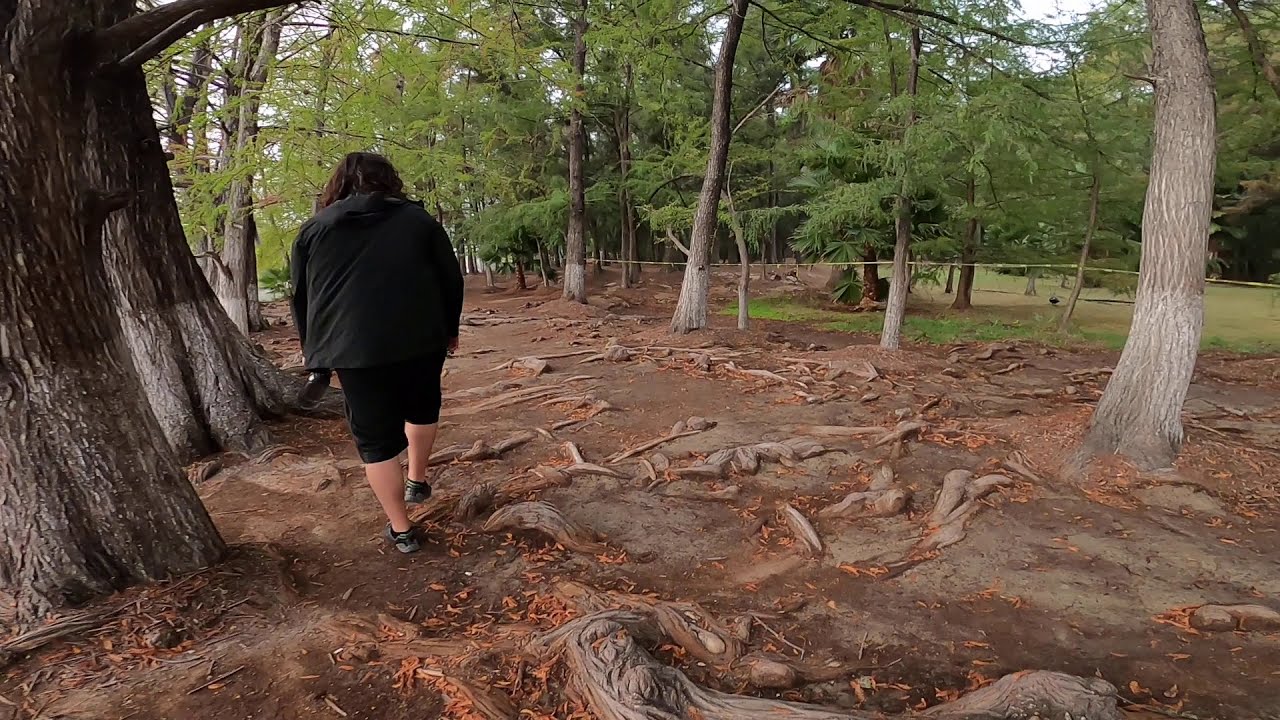This photograph, taken outdoors during daylight, showcases a nature trail likely in a wetland area. The scene features a person walking away from the camera down a dirt path flanked by dense trees on both sides. The person, who has long hair, is clad in a light black, long-sleeved jacket, black shorts, and gray sneakers. They hold an indistinguishable object in one of their hands.

The trail is covered with massive, gnarled tree roots protruding from the earth, suggesting a potentially hazardous walk. The trees, which are especially thick on the left side of the path, exhibit signs of past submersion; their trunks show a distinct, evenly distributed white discoloration, likely indicating previous water levels. Caution tape encircles some trees on the right-hand side in the distance. The sky above is a whitish blue, implying the photo was taken during the day. In the background, there are more trees and patches of grass unaffected by fluctuating water levels, hinting at the area's dynamic environmental conditions.